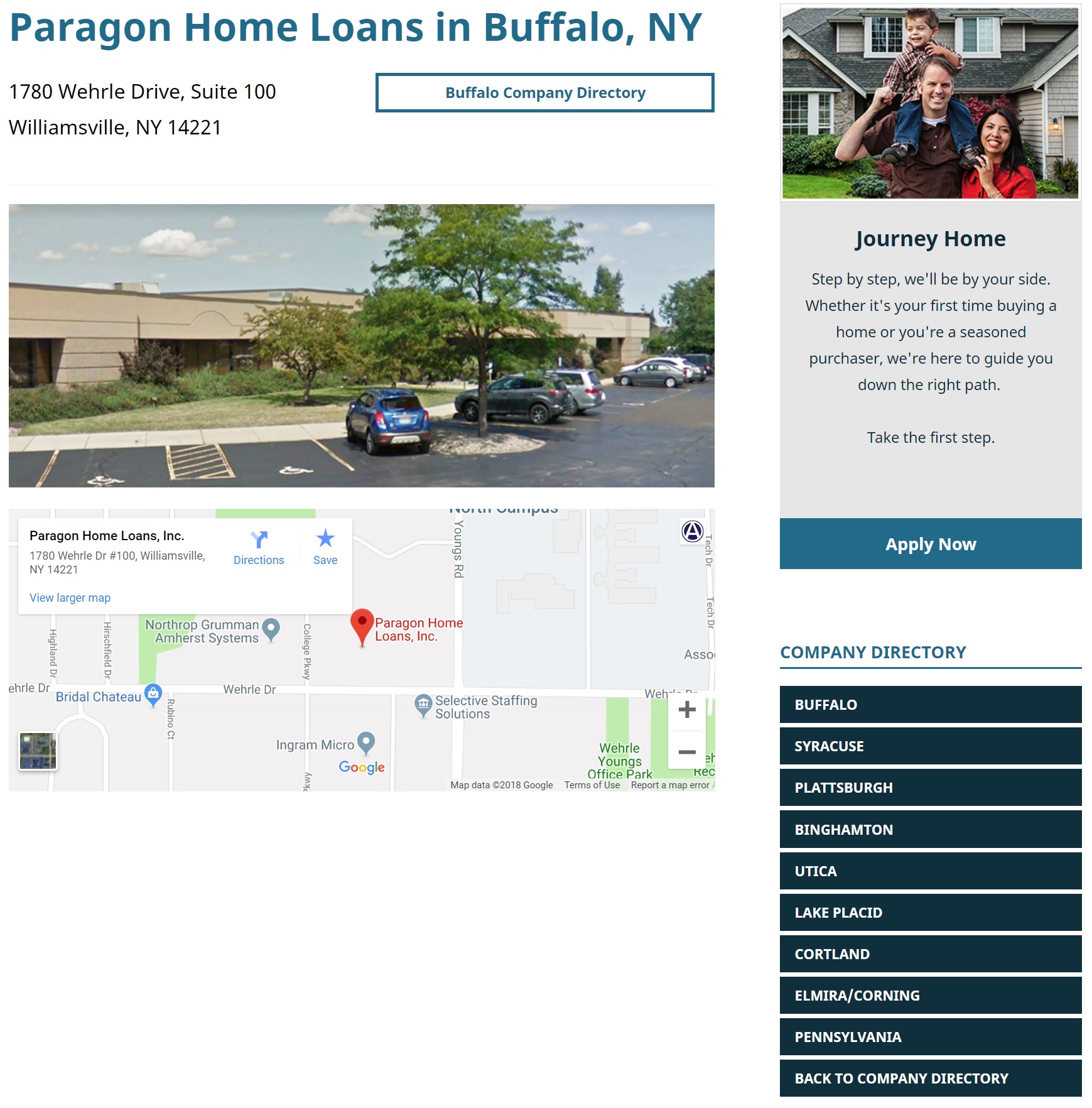The image showcases Paragon Home Loans located in Buffalo, New York. In the upper left-hand side of the image, the company's name is prominently displayed in a larger aqua-colored font. Directly below, the address is listed in black, left-justified font: 1780 WEHRLE Drive, Suite 100, Williamsville, New York, 14221. To the right of this text, there's a Buffalo Company Directory box. Beneath this directory box is a Google Maps image pinpointing the location of Paragon Home Loans, Inc. The right side of the image is dedicated to a section labeled "Journey Home," featuring a heartwarming picture of a man with a child on his shoulders and a smiling woman, all in front of a house. An "Apply Now" button is located at the bottom of this section. Adjacent to this, there's another segment on the right-hand side indicating the Company Directory, providing further details about Paragon Home Loans.